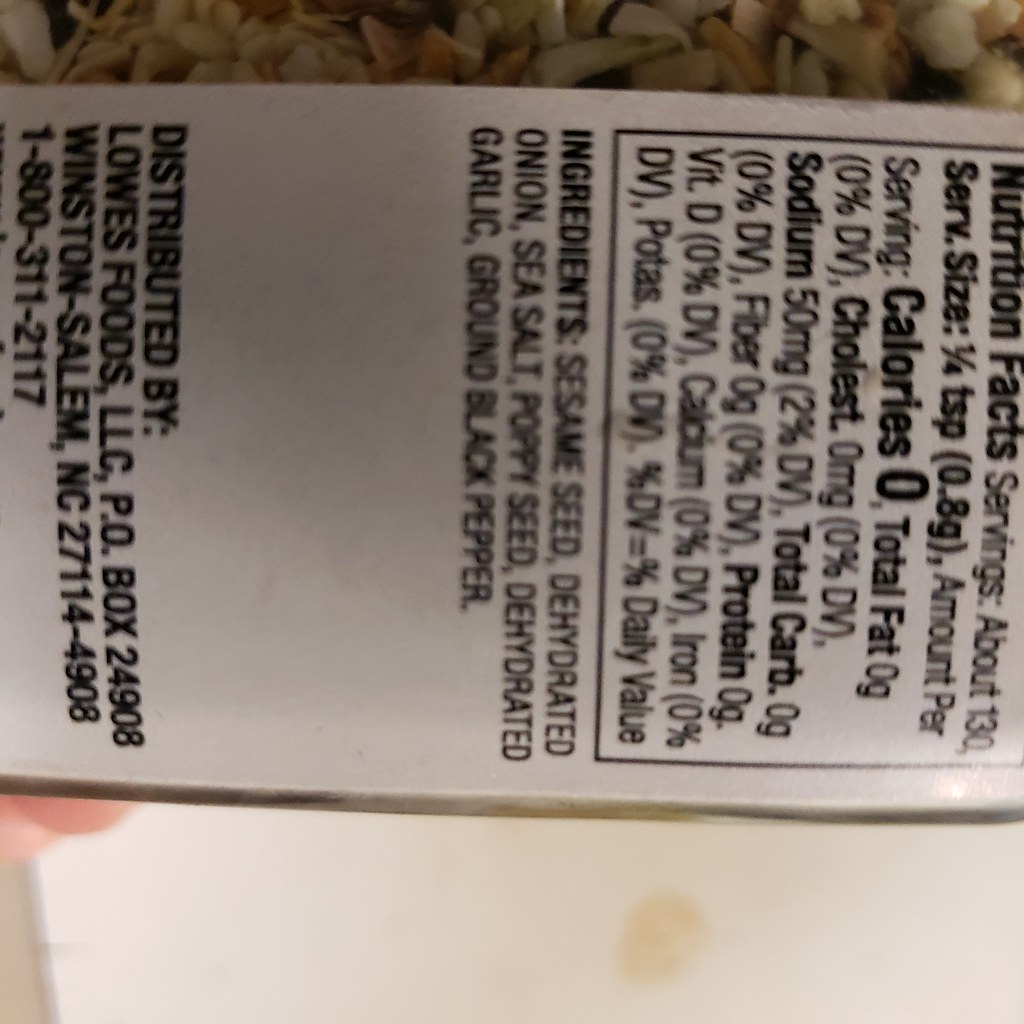This is a slightly blurry but readable photograph taken indoors of a nutrition label on a package of what appears to be a mix of seeds and spices. The white label with black print is rotated towards the right, requiring you to turn your head to read it properly. It details that the product contains about 130 servings, with each serving size being a quarter teaspoon (0.8 grams). The nutritional content per serving includes zero calories, zero fat, zero cholesterol, 50 milligrams of sodium (2% daily value), zero total carbohydrates, zero dietary fiber, and zero protein. The ingredients listed are sesame seeds, dehydrated onion, sea salt, poppy seed, dehydrated garlic, and ground black pepper. The product is distributed by Lowe's Foods LLC, PO Box 24908, Winston-Salem, North Carolina, 27114-4908, with a contact phone number of 1-800-311-2117. The background of the image appears to be a table surface, adding to the context of the indoor setting.